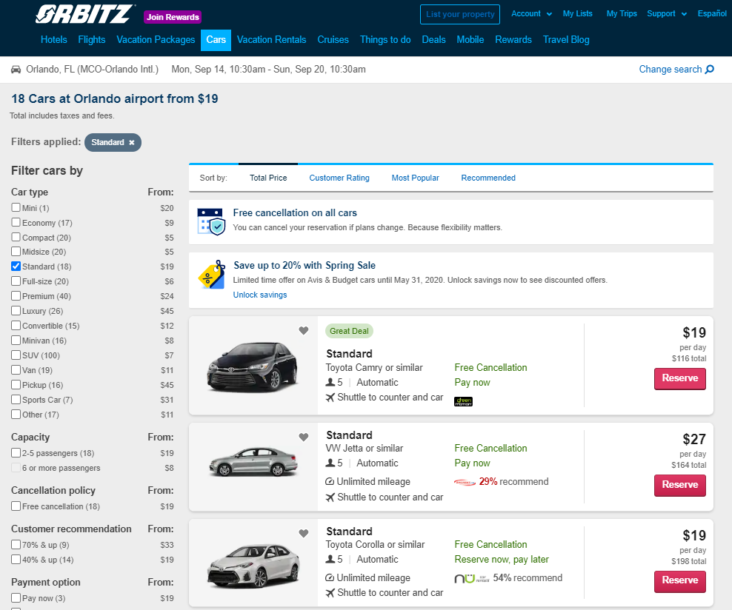Here's a cleaned-up and detailed description of the screenshot from the Orbitz website for car rentals:

---

**Detailed Screenshot Description of Orbitz Car Rental Page:**

The screenshot displays a neatly organized car rental search results page on Orbitz. At the very top, there is a prominent blue menu banner with the Orbitz logo in large white text. Adjacent to the logo is a small, eye-catching purple banner that reads "Join Rewards" in white text. 

Moving along the top menu bar, there are six available options: 
1. "List Your Property" (which is encircled and highlighted)
2. "Account"
3. "My Lists"
4. "My Trips"
5. "Support"
6. "Español"

Directly below this primary menu bar is a secondary row of options. This menu provides 11 different categories for navigation, including:
- Hotels
- Flights
- Vacation Packages
- Cars
- Vacation Rentals
- Cruises
- Things to Do
- Deals
- Mobile
- Rewards
- Travel Blog

Specifically highlighted is the search result for Orlando, Florida (or Orlando International Airport, MCO) alongside the selected dates and times. The title of the section reads, "18 cars at Orlando Airport from $19,” indicating the availability and starting price of rental cars. Standard filters have been applied to these search results.

To the left is a sidebar titled "Filter Cars By," offering options for refining the search:
1. Car Type
2. Capacity
3. Cancellation Policy
4. Customer Recommendation
5. Payment Options

In this sidebar, the only selected filter under "Car Type" is "Standard."

The main search results column presents various car options and is initially sorted by "Total Price." Additional sorting options include "Customer Rating," "Most Popular," and "Recommended."

A banner below the sorting options features a small calendar icon with a checkmark, stating, "Free cancellation on all cars," followed by a concise description of this benefit. Further down, another banner, titled "Save Up to 20% with Spring Sale," includes receipt tags and a link with blue text, "Unlock Savings."

Displayed in this section are three prominent car rental options:
1. **First Car:**
   - Appearance: Dark two-door car under the "Standard" category
   - Highlights: "Great deal," free cancellation
   - Price: $19 per day, $116 total
   - Action: "Reserve" button

2. **Second Car:**
   - Appearance: Side shot of a light-colored four-door sedan
   - Details: Automatic or manual transmission options, unlimited mileage
   - Price: $27 per day
   - Action: "Reserve" button
   - Cancellation: Free

3. **Third Car:**
   - Make: Standard Toyota Corolla
   - Price: $19 per day
   - Action: "Reserve" button
   - Cancellation: Free

These options are presented clearly with visuals and actionable buttons to facilitate the reservation process.

---

This description provides a detailed and structured caption of the screenshot, giving a comprehensive overview of the information displayed on the Orbitz car rental page.